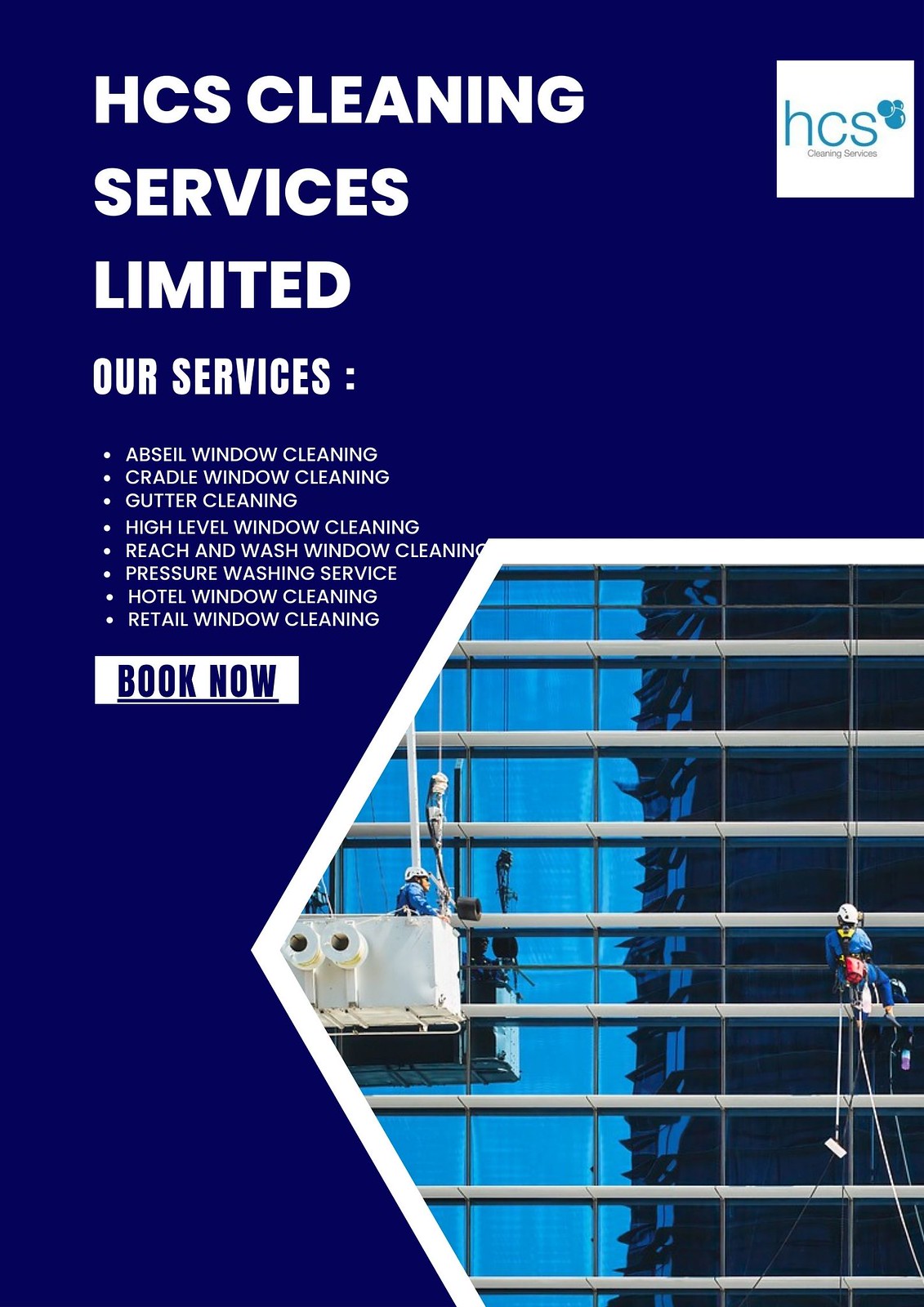The image depicts a promotional material for HCS Cleaning Services Limited. In the top left corner, white text on a dark blue background reads "HCS Cleaning Services Limited," followed by "Our services:" and a list of bullet points advertising various cleaning services: Absolute Window Cleaning, Cradle Window Cleaning, Gutter Cleaning, High Level Window Cleaning, Reach and Wash Window Cleaning, Pressure Washing Service, Hotel Window Cleaning, and Retail Window Cleaning. A small white rectangle with a dashed line underneath says "Book Now." 

In the top right corner, there is a small white square containing a blue logo and the text "HCS Cleaning Solutions."

The central image, shaped as part of a hexagon, shows two professional window cleaners working on a very tall building. One worker, wearing a safety helmet and blue shirt, stands in a movable elevator-like box, while the other, suspended by ropes and harnesses, is positioned nearby with a white bucket. The image captures the high-risk and meticulous nature of their job.